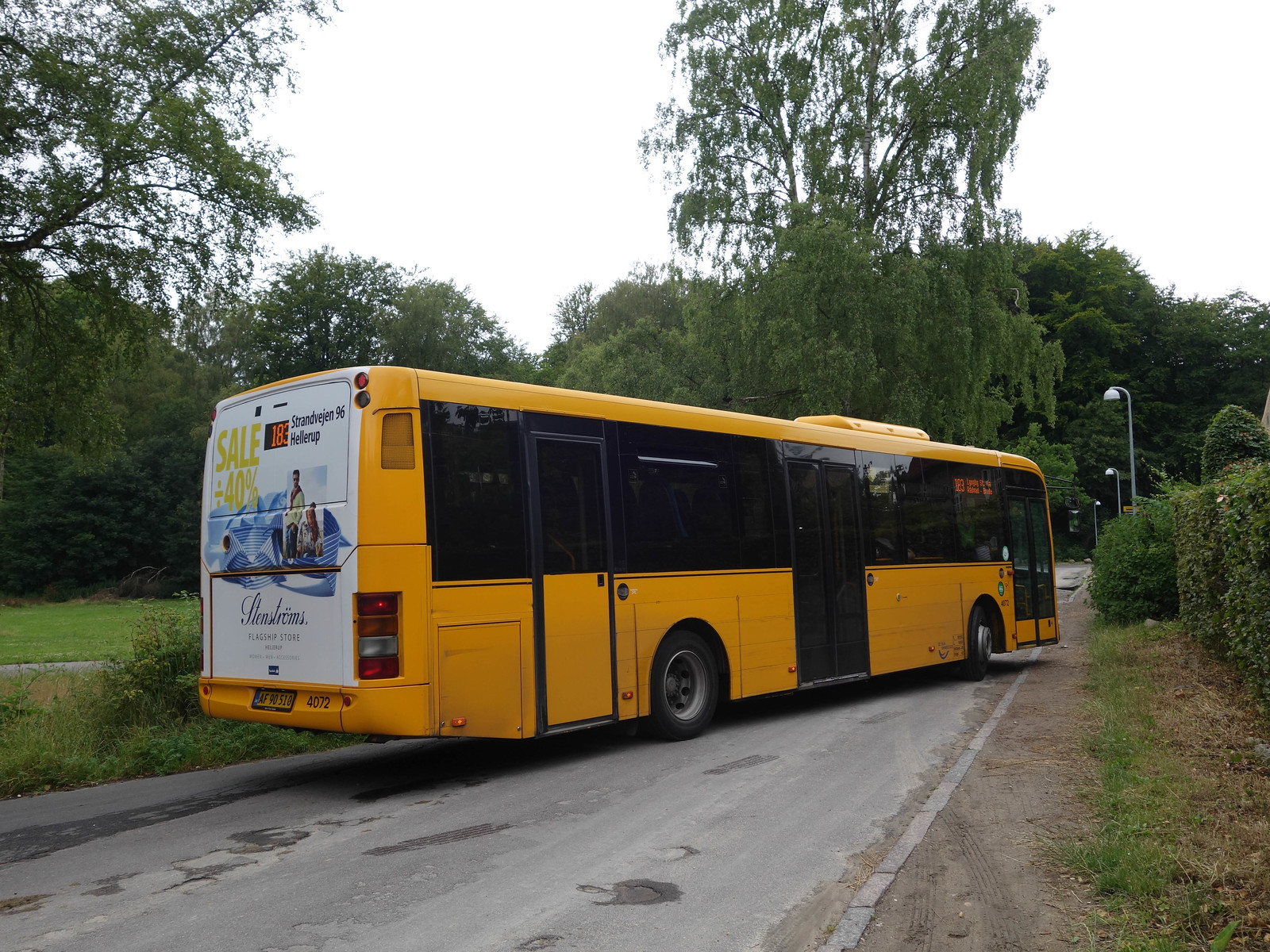This image depicts a very long yellow bus, reminiscent of a city bus yet painted in the distinct yellow color commonly associated with school buses. The bus, unusually large with multiple doors and sleek frameless black windows, is positioned diagonally across a small, lightly trafficked road, almost entirely blocking it. The road appears worn and poorly maintained, with visible potholes, cracks, and scuffed pavement. The bus features illumination from a destination sign on its side and is adorned at the back with a semi-blurry advertisement promoting a 40% sale from "Strandmeier" or a similarly-named brand, partially written in a language that seems Dutch or Swedish.

Surrounding the bus, the area includes grassy patches, low bushes, and a line of silver streetlights with yellow bulb covers extending into the distance. To the left, there's a scenic park area or possibly an amusement park, indicated by green pathways and numerous trees. More trees and plants border the road, contributing to the impression of a semi-rural or park setting. The sky in the background is overcast or very light, giving it an almost white appearance. 

Additional details include the bus's yellow license plate marked "AF90510," rear route number signage indicating either Route 183 or 4072, and distinctive black tires with silver rims. The bus, which has buttons next to each door for opening, seems either to be caught mid-maneuver or awkwardly parked, with no visible pedestrians or bus occupants discernable in this particular shot.